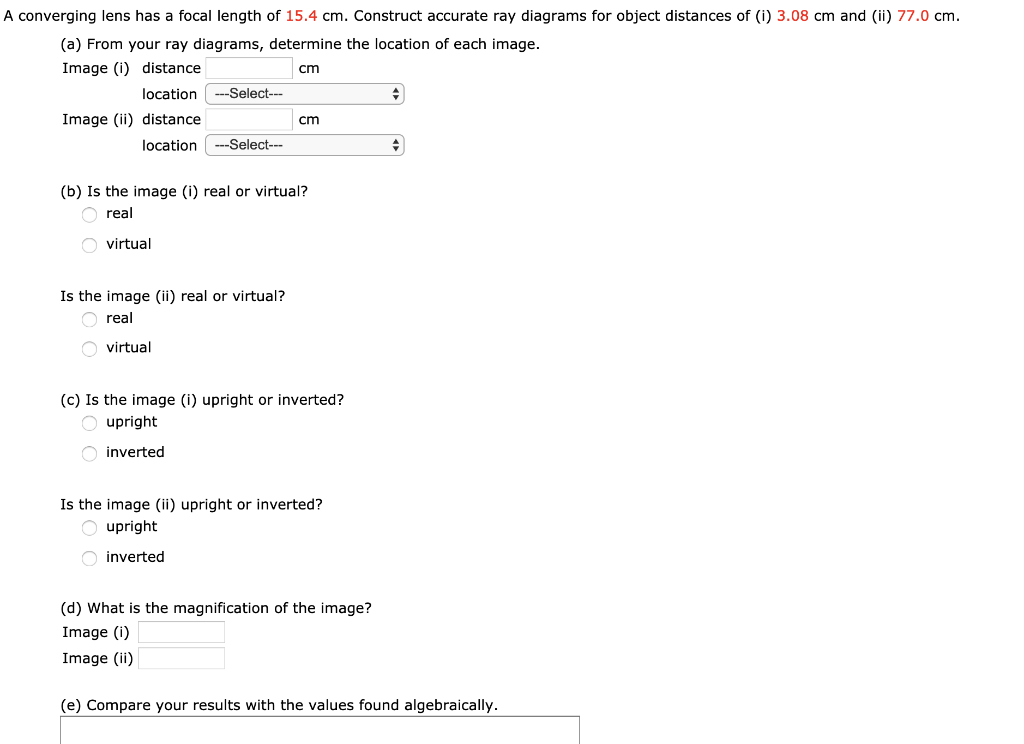Image caption: Detailed instructions are provided for constructing accurate ray diagrams using a converging lens with a focal length of 15.4 cm. The task involves plotting ray diagrams for object distances of 3.08 cm and 77.0 cm to determine the locations of each respective image. The instructions prompt users to identify the following: 

A. Calculate the precise location of Image 1 and Image 2, referring to the specific distances in cm. 
B. Determine if each image is real or virtual, prompting a selection between the two options for both images. 
C. Ascertain whether each image is upright or inverted. 
D. Calculate the magnification of each image accurately. 
E. Compare the diagram results with the values derived algebraically.

This comprehensive task ensures a thorough understanding of ray diagrams and lens behavior through hands-on practice and analytical comparison.